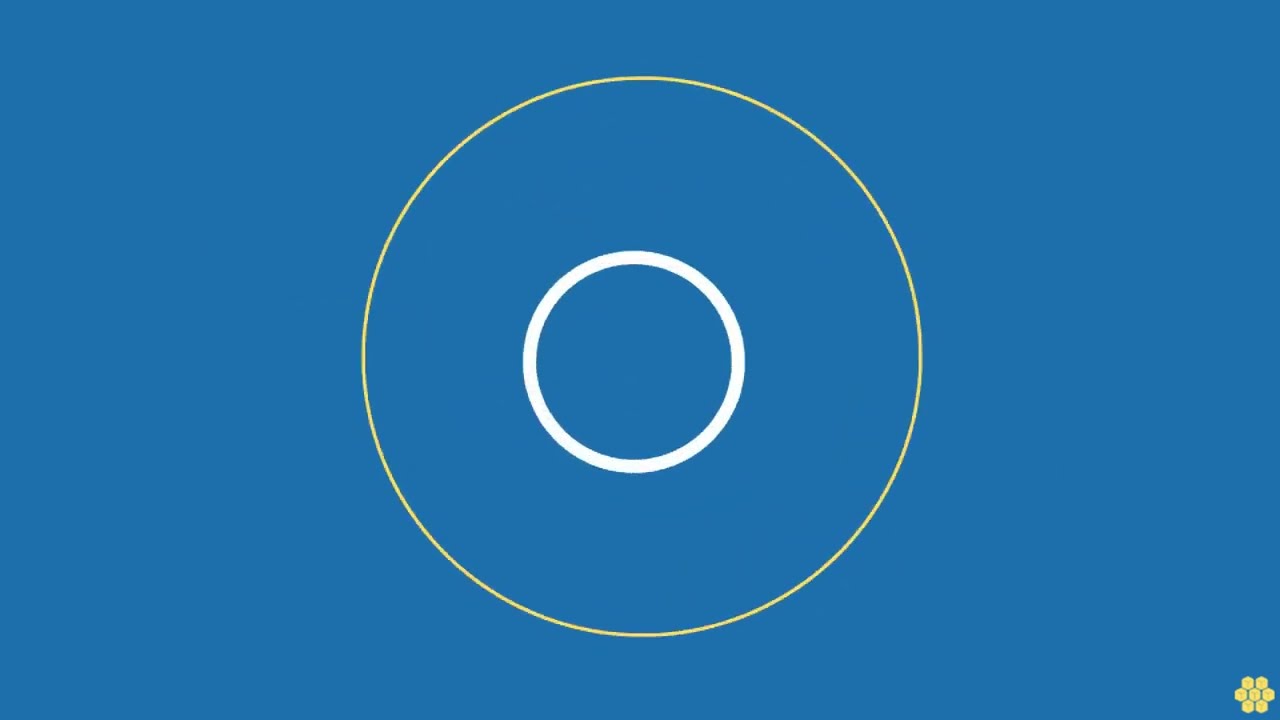The image features a blue rectangular background with a slightly grayish tinge, wider than it is tall. In the center, there is a series of concentric circles: an inner white ring approximately 1.5 units in diameter, surrounded by a thinner yellow ring that is roughly three times the diameter of the inner circle. Both rings are centered within the image. Toward the bottom right corner, a small yellow honeycomb pattern is visible, consisting of seven hexagonal shapes—arranged with two hexagons on the top row, three in the middle, and two on the bottom row. This honeycomb symbol is much smaller in comparison to the rings and could fit multiple times within the white circle. The overall design is minimalistic, without any text or additional elements.